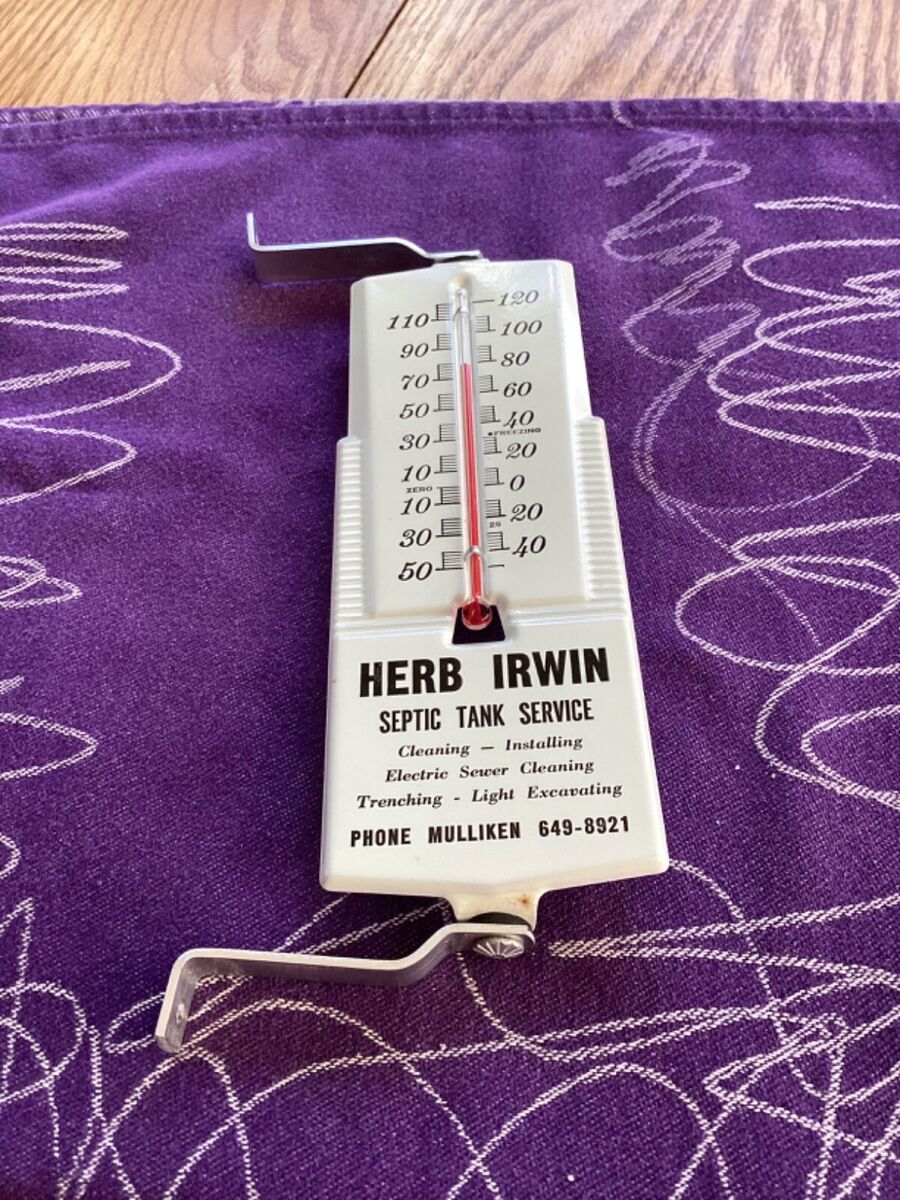The image depicts a vibrant purple blanket adorned with white squiggly lines, positioned atop a wooden surface that is partially visible in the upper section of the photograph. Resting on the blanket is an antique-style metal thermometer, featuring a white facade with dual temperature scales – Fahrenheit on one side and Celsius on the other – that measure from 120°F (50°C) downwards. The thermometer is equipped with metal brackets at both the top and bottom for mounting purposes. Central to the device is a glass rod with a bulb at the end, indicative of its functional design for temperature measurement. Prominently, the base of the thermometer is marked with the branding and services of "Herb Irwin Septic Tank Service," including details such as "Cleaning Installation Electric Sewer Cleaning Trenching Light Excavating," along with the contact number "649-8921". This promotional thermometer, likely distributed as an advertisement by the business, contrasts with the striking purple of the blanket which initially captures attention in the image.